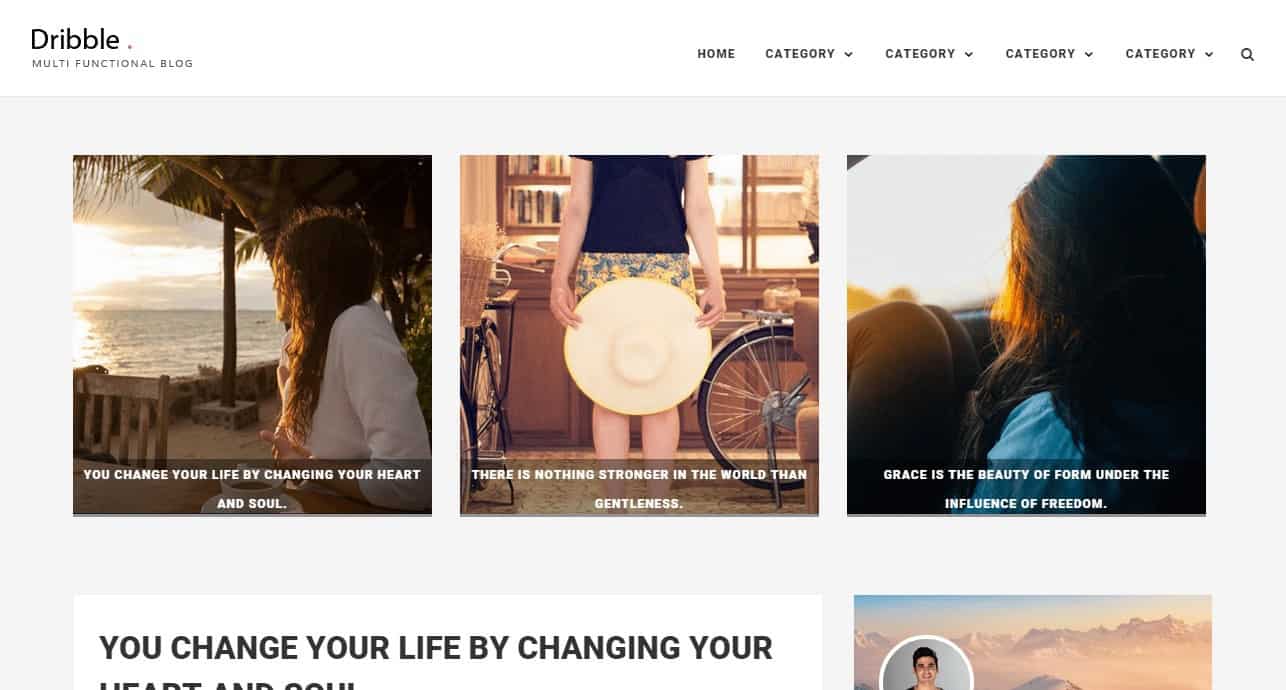Detailed Description of the Landing Page Mock-Up:

The landing page mock-up features a clean layout with varied imagery and text elements. At the top, set within a white bezel, the word "Dribble" is prominently displayed in black text, with the first 'D' capitalized. Below it, in bold gray text, is the phrase "Multi-Functional Blog."

On the right side of the navigation bar, there are several tabs in all caps and bold black text. The first tab reads "HOME," followed by multiple instances of "CATEGORY" with drop-down arrows. The final element on the right is a magnifying glass icon, indicating search functionality and hinting that the mock-up is not fully edited.

On the left side of the page, an image shows a woman with shoulder-length brown hair gazing out at an ocean. The ocean scene features a large yellow sun and spans into dark gray clouds with hues of yellow cascading down. There are gray stones of varying shades, a brown overhang, and a dark green palm tree. The woman, dressed in a long-sleeve white shirt, is accompanied by bold white text that says, "You change your life by changing your heart and soul."

Another section of the page presents an indoor scene, resembling a kitchen, where a woman stands or sits between two vintage-style bikes. The bikes are equipped with silver guards and one features a round wicker basket, filled with bundles of light tan wheat. Behind her, a bookcase filled with books of various colors, including white and brown, is visible against a clear window and a white wall. The woman's attire includes a dark blue shirt and a yellow skirt with dark blue splotches. Her lower body is shown without revealing her face, and she is Caucasian. The room's floor is tan and brown, with sunlight streaming in. Bold white text beneath this image reads, “There is nothing stronger in the world than gentleness.”

On the right side, another image shows a woman with shoulder-length black hair, sitting with her knees to her chest, dressed in black leggings and a jean jacket blue shirt. She gazes out at a dark gray sky with trees in shades of yellow and light green. Overlaid on this image is white text that reads, “Grace is the beauty of form under the influence of freedom.”

A partially visible white rectangle on the left side of the page contains bold black text stating, "You change your life by changing your heart and soul," though some words are cut off. Adjacent to it, a white circle with a dark gray interior features an individual with round hair and Caucasian skin. The backdrop presents a dark blue sky with streaks of white, along with white mountains tinged with pink and hot pink peaks, adorned by thin fog-like white clouds.

This meticulously detailed layout combines striking visual elements, varied typography, and motivational text to create an engaging and versatile blog landing page mock-up.